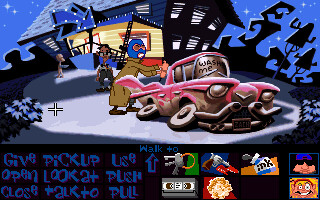This square-shaped graphic artwork is teeming with intricate details, centering around a prominently featured pink car. The car, depicted with two side doors and visible front window wipers, bears text on its front window. Intriguingly, the wheels of the car appear deflated and sideways, adding a surreal touch. Behind the car stands a figure wearing a blue mask and a long, brown coat, emanating a mysterious presence. The scene is set against the backdrop of a yellow house, which adds a contrasting layer of vibrancy to the overall composition.